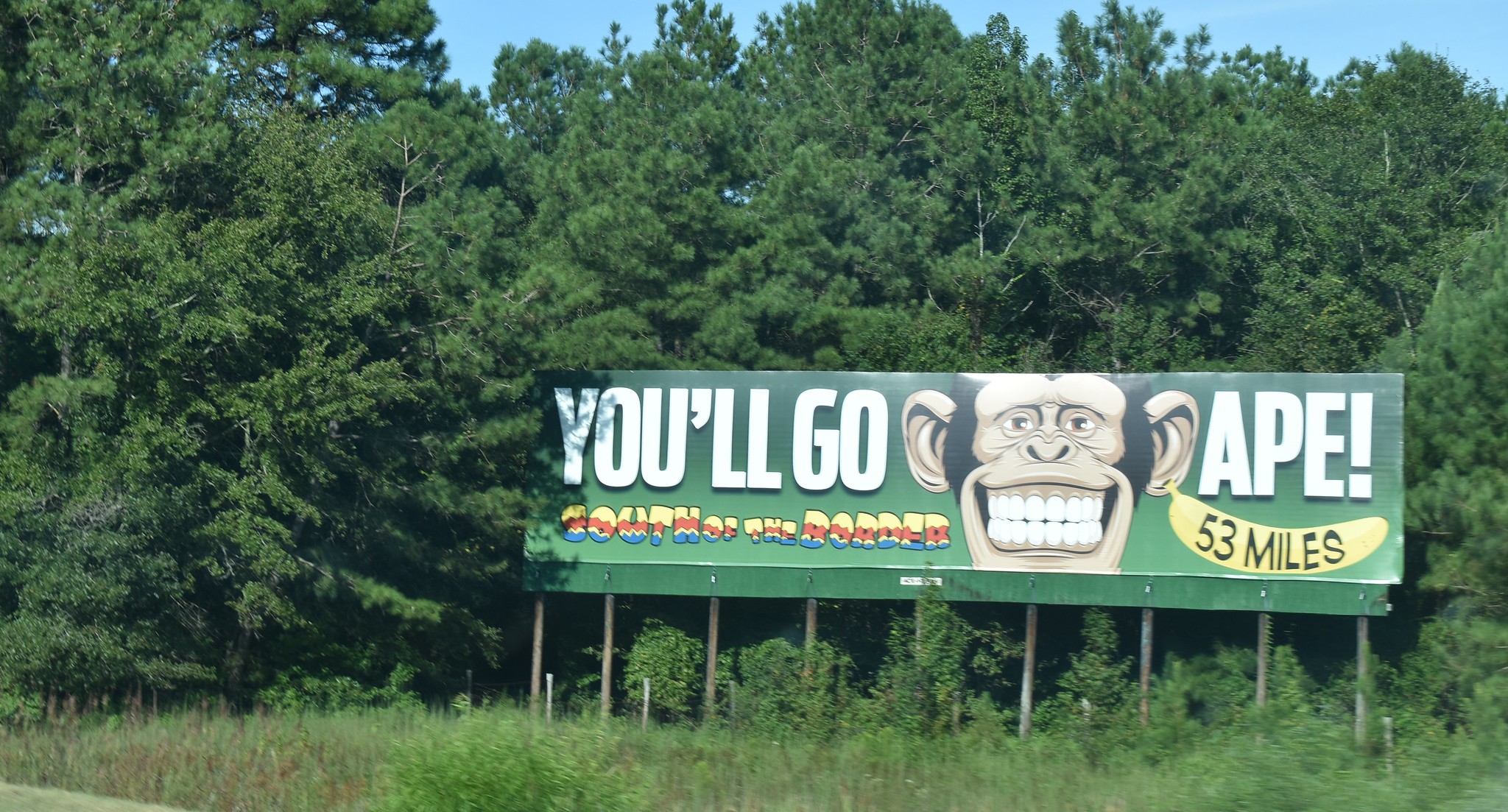This color photograph features a large, rectangular billboard held up by several gray poles. The sign has a green background with the phrase "You'll Go Ape" displayed in white illuminated letters. Centrally placed between the words "Go" and "Ape" is a cartoon image of a smiling monkey, revealing both rows of its gritted teeth. On the left, just below the main slogan, additional lettering reads "South of the Border," designed in a whimsical, cartoony style with yellow at the top, red in the middle, and blue at the bottom. On the right side, there is an illustration of a banana with "53 miles" written in black on it.

In the background, the upper part of the image features a blue sky, with patches visible above the dense tops of fir trees, resembling Christmas trees. Below the sign, mixed greenery including bushes, tall grasses, and brownish weeds extends across the width of the foreground. The scene captures a blend of natural and advertising elements in a vivid outdoor setting.